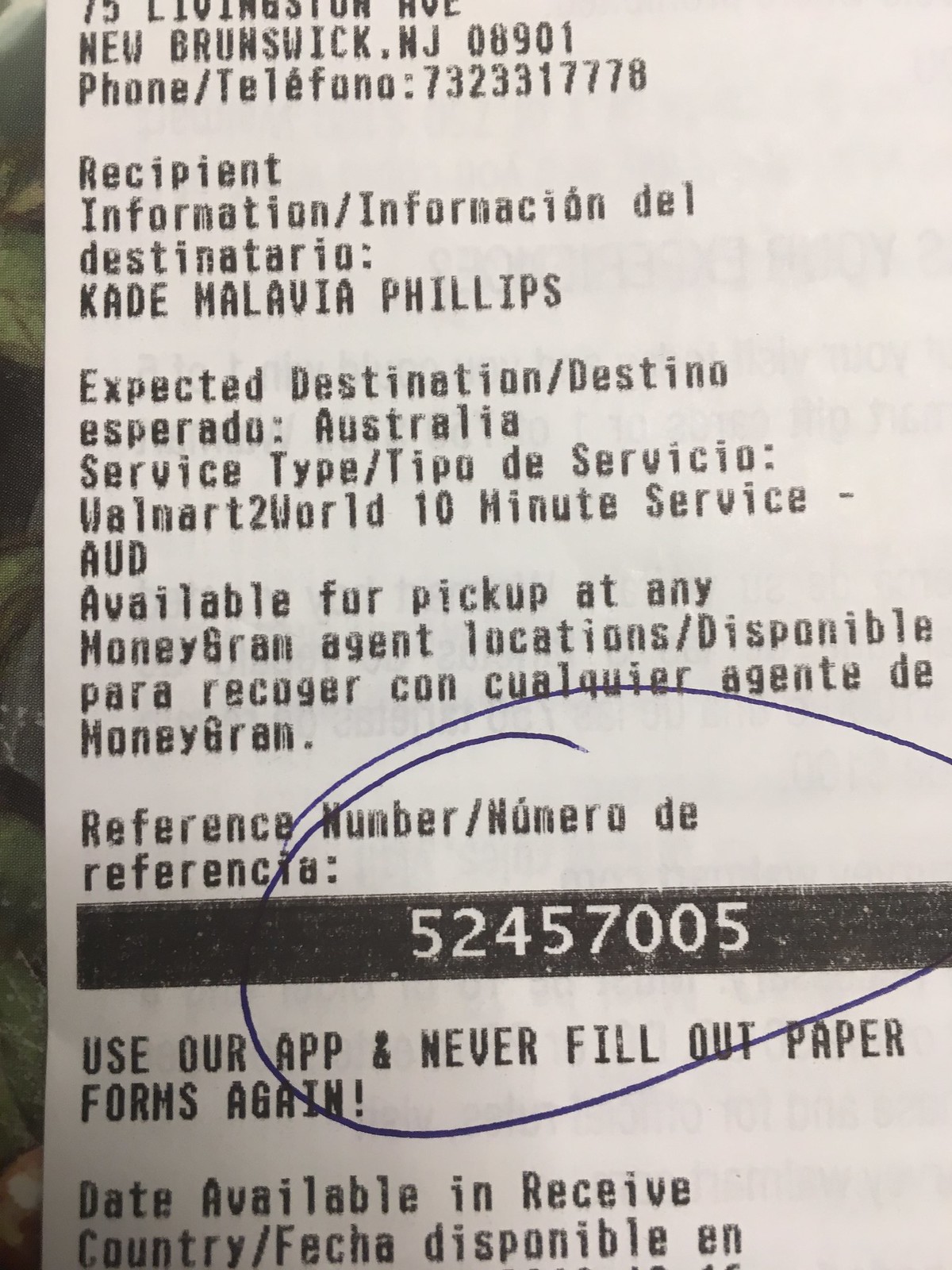A close-up image of a partially cut-off receipt sits atop a lightly visible tablecloth that peeks through on the left-hand edge of the frame. Dominating the image is the receipt, where the top segment is slightly truncated, revealing just enough to make out "New Brunswick, New Jersey 08901" and a partial phone number. Scattered text on the receipt includes phrases like "expected destination" and "Australia," suggesting it might be for a ticket or a MoneyGram transfer. Notably, a phrase stating "Available for pickup at any MoneyGram" is legible. Toward the bottom center of the receipt, a blue circle encloses a black bar printed with the number "524-57005," emphasizing its significance.